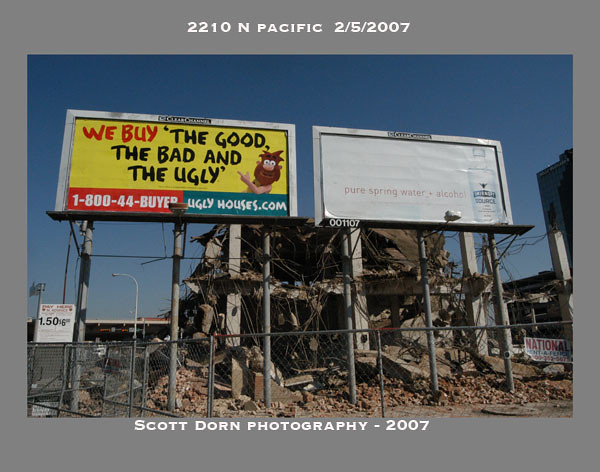This photo, dated February 5, 2007, captures the address at 2210 North Pacific. Prominently featured are two billboards: one advertising a company that buys houses in any condition with the slogan "We Buy the Good, the Bad, and the Ugly" and a contact number 1-800-44-BUYER, followed by the URL 'UGLY-HOUSES.COM.' The second billboard promotes Smirnoff vodka, highlighting "Pure Spring Water Plus Alcohol." The bottom of the image credits "Scott Dorn Photography 2007." In the background, there is a heavily damaged building, appearing to be in a state of serious disrepair.